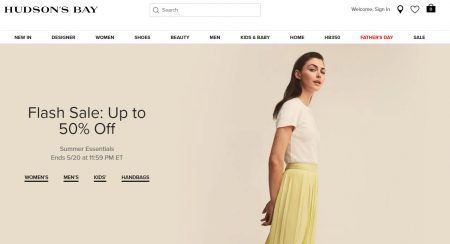The image is a rectangular screenshot taken from the website of Hudson's Bay. In the upper left corner, the company’s name "Hudson's Bay" is prominently displayed in black font against a white background. Below the company name, there are several clickable sections in bold black text designed to help users navigate different parts of the website. Notably, the second link from the right is displayed in red font, suggesting it has been activated or selected.

Toward the bottom of the image, there is a large rectangular advertisement prominently featuring a flash sale offering up to 50% off. Below this offer, a promotional code is provided in a very dark red color, bordering on black or gray but with a hint of red. 

On the right side of the advertisement is a photograph of a young girl with medium-length black hair slicked back, cascading down her back. She is dressed in a white t-shirt paired with what appears to be loose-fitting light yellow pants or a possibly wrinkled long skirt, belted at the waist. The background she is standing against features soft hues of light yellow and pink, giving the image a warm, inviting feel.